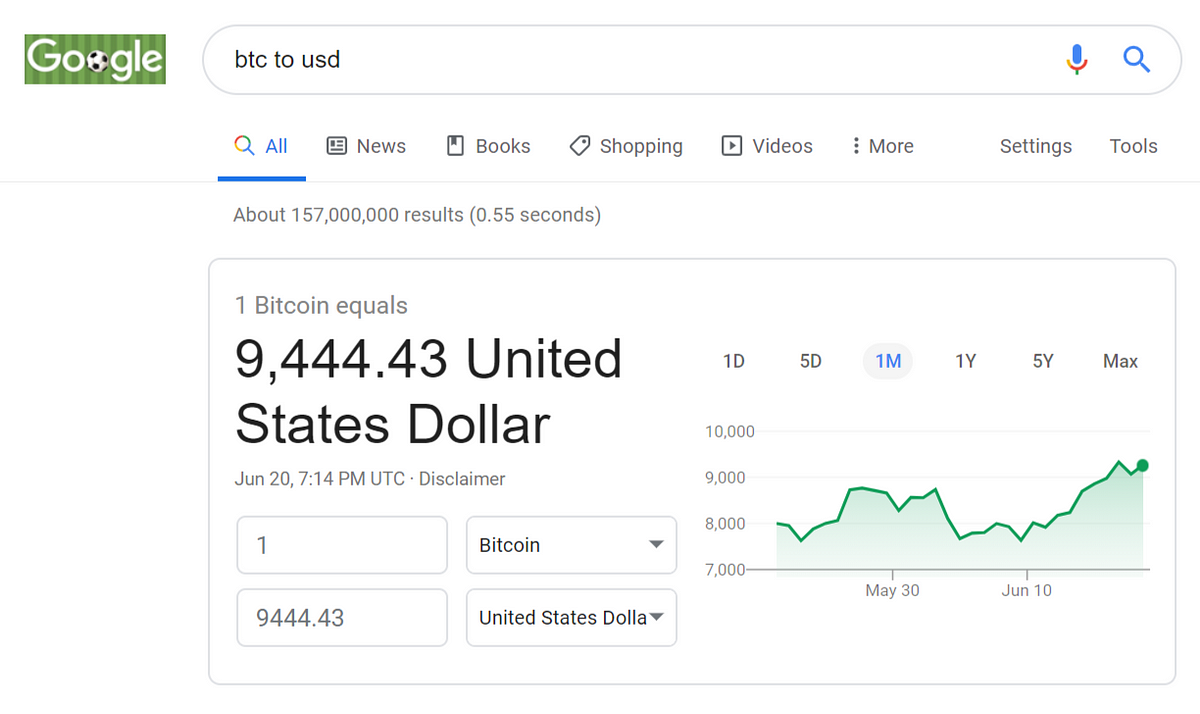The image displays a Google search results page specifically for converting Bitcoin to United States Dollar (BTC to USD). In the top-left corner, the Google logo is visible, resembling the layout of a soccer field. Below the logo is a search bar containing the text "BTC to USD," accompanied by a microphone icon. The navigation bar underneath includes links labeled "All," "News," "Books," "Shopping," "Videos," "More," "Settings," and "Tools."

Displayed prominently is a chart tracking the value of Bitcoin over time. The conversion rate highlighted at this moment shows Bitcoin valued at $9,444.4396. The page mentions approximately 157 million search results returned in 0.55 seconds. The chart further details Bitcoin's fluctuation, starting at $8,000, and its movement over different periods such as 1 day, 5 days, 1 month, 1 year, 5 years, and maximum timeline available. Significant points on the chart include data from May 30th where Bitcoin was oscillating between $9,000 and $8,000, June 10th when it dipped below $8,000, and its subsequent rise to the current value of $9,444.

Additionally, the interface includes drop-down menus allowing the user to select Bitcoin and U.S. Dollar, with options to compare other currencies. The chart visually represents these currency conversions and fluctuations over specified time frames.